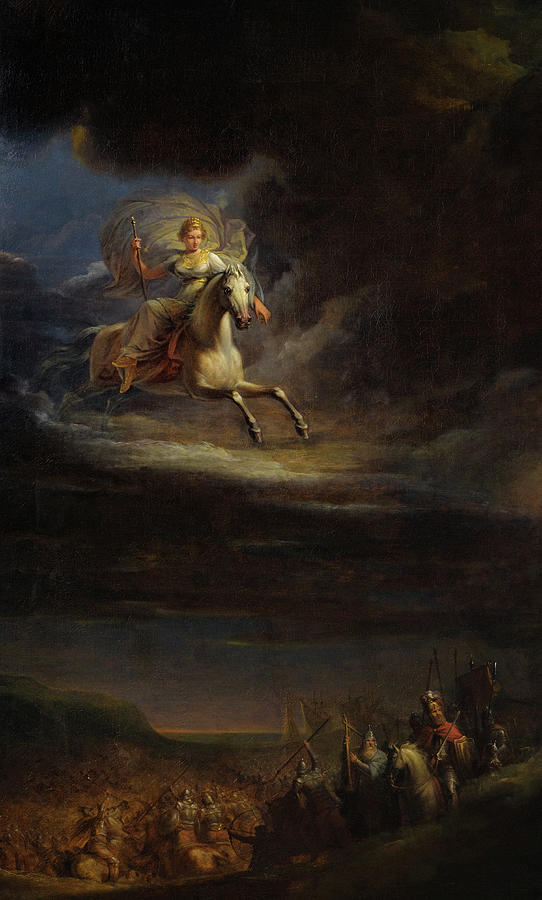In this fantasy watercolor painting, a dramatic battle scene unfolds under a dark, stormy sky. The image is filled with armored soldiers on horseback and on foot, wielding spears and standing on a hillside. Their armor glints with dark accents and various shades of red and blue peek through their battle attire. Amidst the chaos of the battlefield, the landscape in the valley stretches out, possibly hinting at a distant castle or ships, shrouded in the mist of war.

Dominating the scene is a woman riding a majestic white horse high in the sky. She exudes an ethereal presence, wearing a long, flowing chiffon gown trimmed in gold, which billows around her like the wings of an angel. A gold crown rests upon her head and she holds a mysterious staff or rod. Her illuminated figure contrasts starkly against the ominous black and gray clouds, the only bright spot in the otherwise dark and menacing scene. Notable is her commanding yet serene demeanor as she gazes down upon the turmoil below, appearing either as a guardian angel or a divine force overseeing the battle.